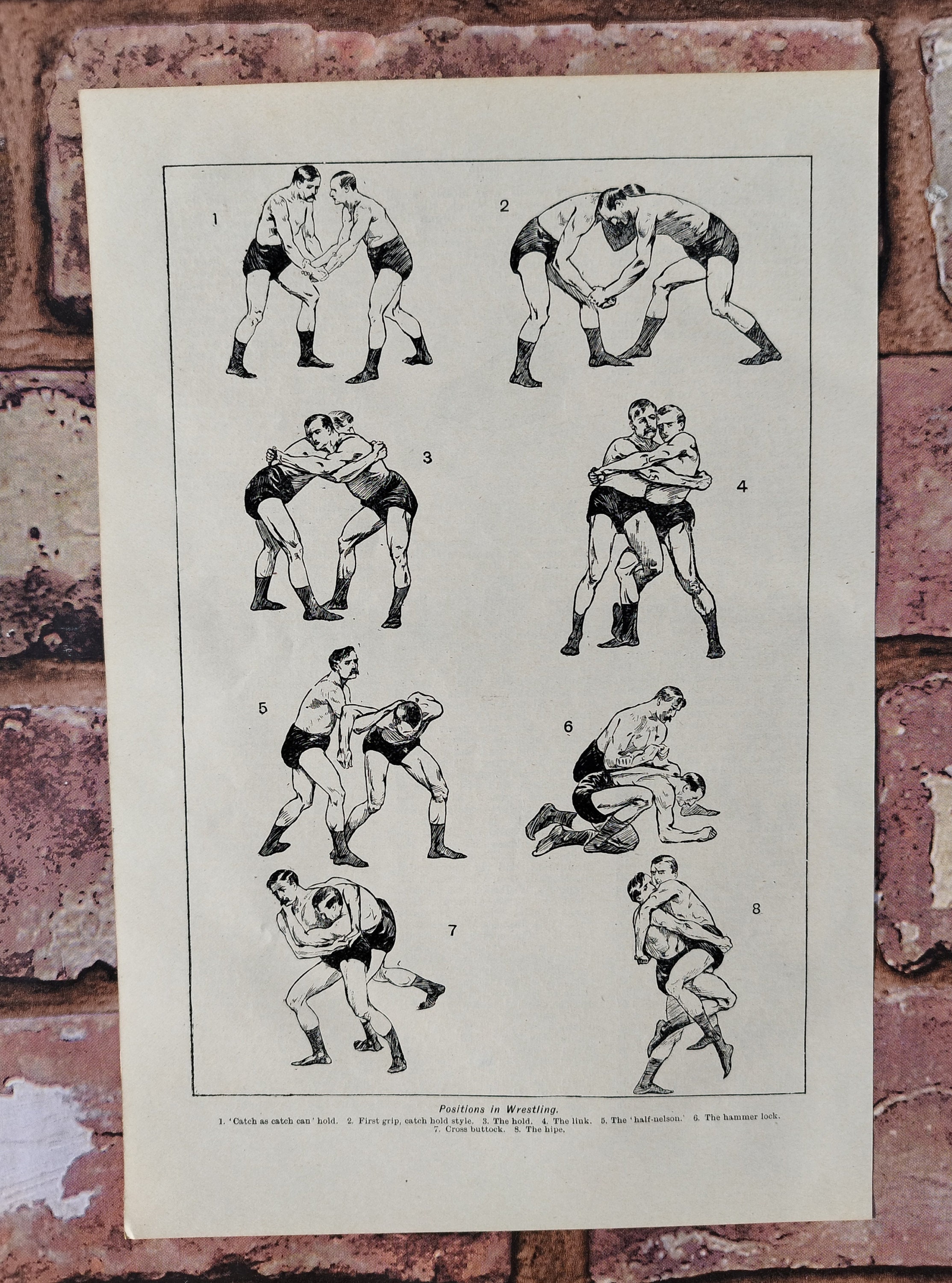This image depicts an old, weathered poster or instructional paper mounted on a rusted red brick wall, illustrating eight sequential steps of a wrestling demonstration conducted by two male individuals. The poster, marked by its dated appearance and featuring men with period-specific haircuts and uniforms, systematically guides viewers through various grappling positions. Starting from the initial stance and progressing through to the eighth step, each stage is meticulously detailed, demonstrating the buildup to the final wrestling position where the wrestlers lock each other firmly in place. Small, hard-to-read print at the bottom likely provides titles and instructions for each step, adding to the instructional nature of the poster.